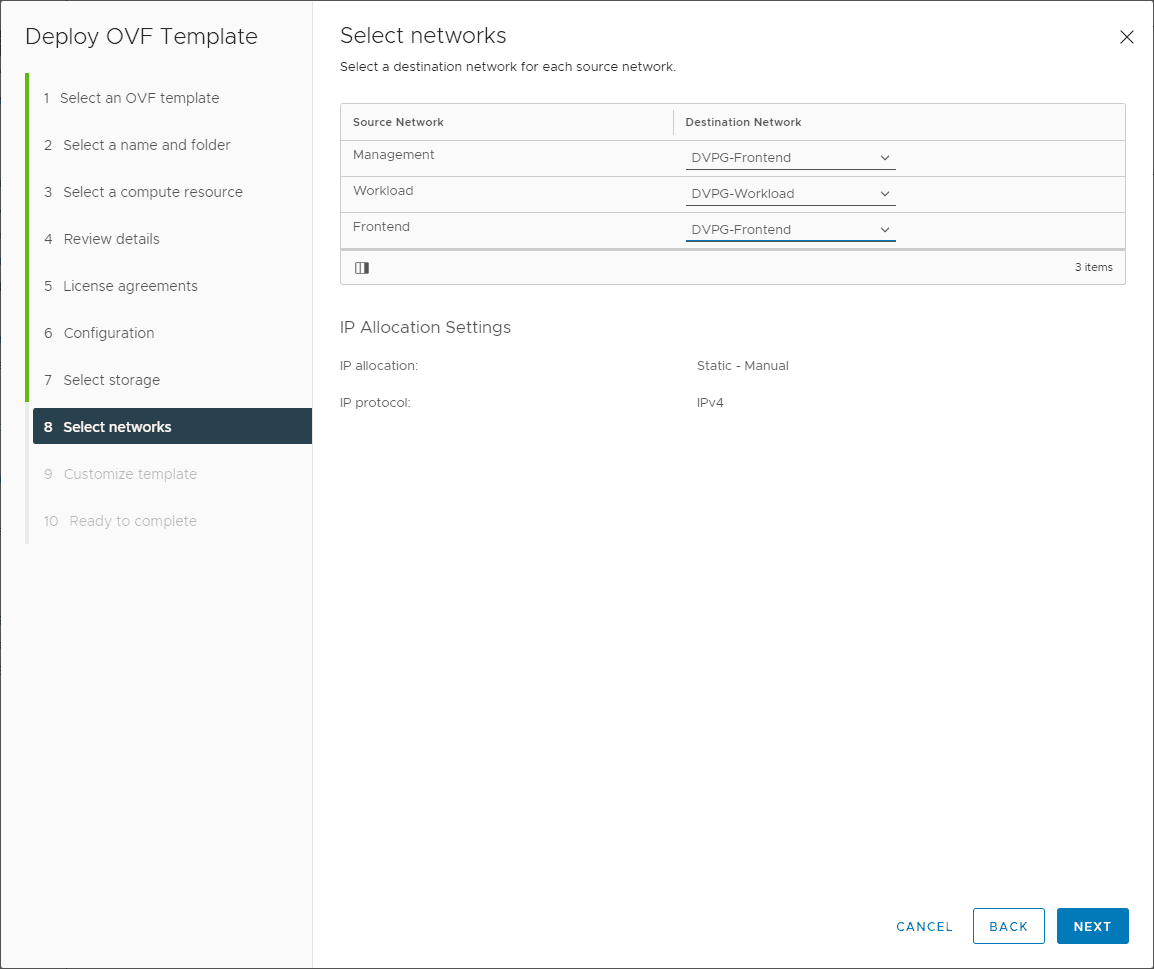**Descriptive Caption: Detailed Breakdown of the "Deploy OVF Template" Screenshot**

The screenshot titled "Deploy OVF Template" is divided into two primary sections on a white background. On the left side is a navigational menu numbered 1 through 10, guiding the user through the deployment process. The steps are as follows:
1. Select an OVF Template
2. Select a Name and Folder
3. Select a Compute Resource
4. Review Details
5. Accept License Agreements
6. Configuration
7. Select Storage
8. Select Networks (currently highlighted)
9. Customize Template
10. Ready to Complete

The main section on the right, labeled "Select Networks," prompts the user to designate a destination network for each source network. This section includes a rectangular table with two columns: "Source Network" and "Destination Network." The listed source networks are "Management," "Workload," and "Frontend." Under the "Destination Network" column, each source network has a drop-down menu offering selections such as "DVPG Frontend" and "DVPG Workload," with additional options that are not visible in the screenshot.

Below this table, the section titled "IP Allocation Settings" appears. It details the following configuration:
- **IP Allocation**: Static Manual
- **IP Protocol**: IPv4

This organized layout provides a clear and detailed interface for deploying the OVF template by specifying network mappings and IP settings.